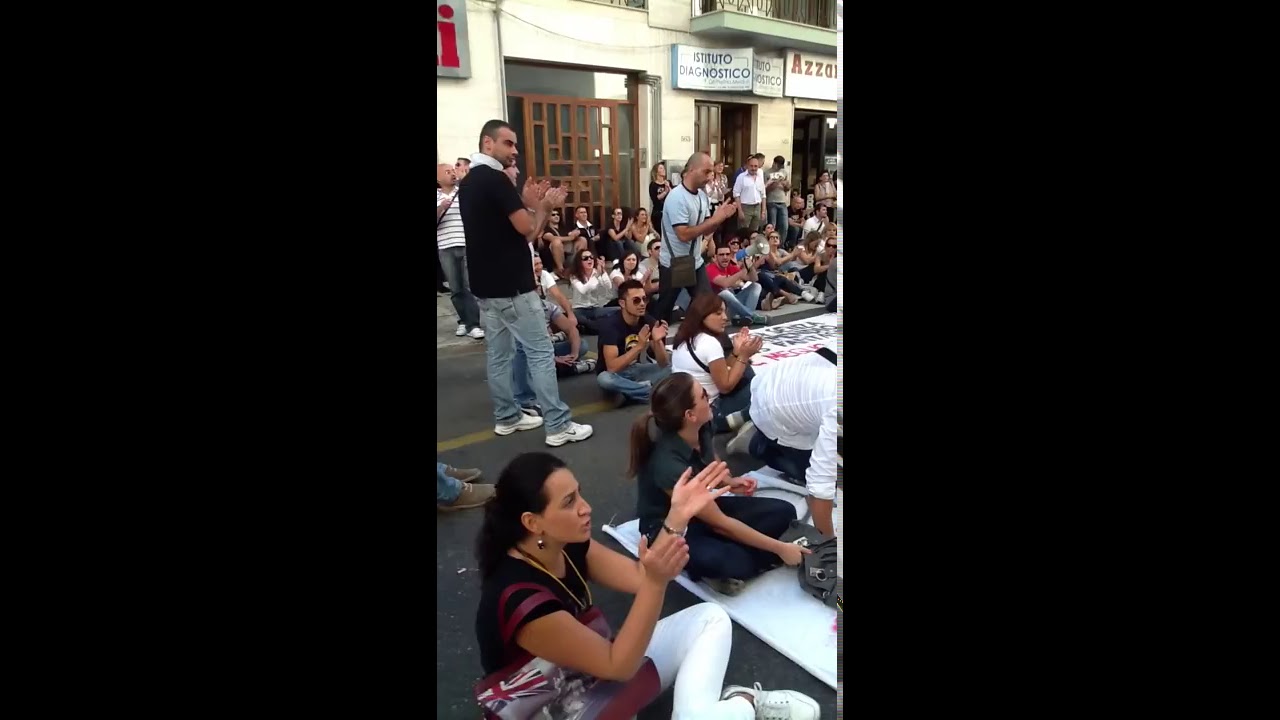The image captures a lively street scene in Italy, densely populated with people focused on a central stage, applauding a performance. The crowd is a mix of younger and middle-aged individuals, sitting mostly Indian-style on the ground, with a few standing and walking around. Dominantly in the foreground is a woman in a black blouse with a handbag over her shoulder, black hair, and white pants. Nearby stands a man in blue jeans, sneakers, and a dark shirt. The backdrop includes white buildings with signage, including Italian text, and a latticed wooden door to a storefront. The atmosphere is vibrant and energetic, characterized by applause and engaged attention towards an unseen performance around the 3:30 position.